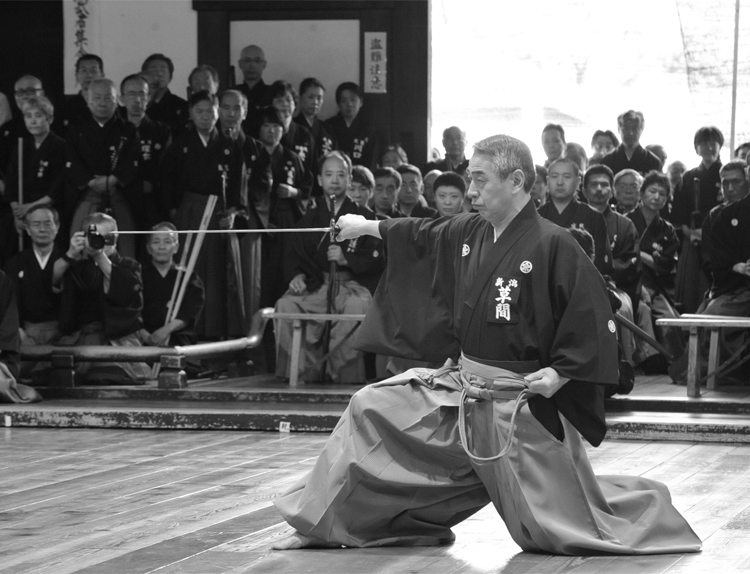A black-and-white photograph captures a man kneeling on a light-colored wooden floor, poised with a silver sword held horizontally. He's dressed in traditional martial arts attire, featuring light-colored, baggy pants fastened with a rope and a black robe-style shirt adorned with white lettering. His stance is precise: one knee is bent forward while his other leg rests on the ground, his calf flat. With a serious expression, he gazes intently into the distance, embodying intense focus. Behind him, a vast audience of at least 30 people is seated, watching attentively. The entire scene exudes a sense of formal martial arts performance or demonstration.